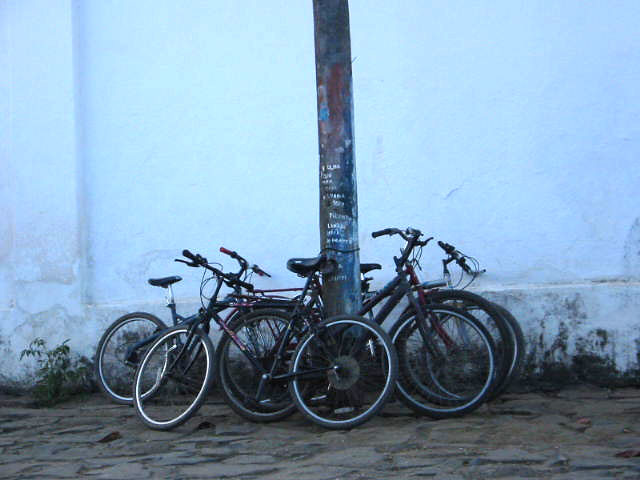This is a bright, outdoor daytime photograph showing a street scene centered around a utility pole with graffiti, surrounded by approximately six or seven classic style bicycles. These bicycles, primarily blue and red in color, are leaning against or chained to the pole, situated on a chipped, cobblestone-paved road or sidewalk. The scene is framed by a textured, bright white building wall, with some foliage growing at the base where it meets the pavement. Despite its semi-focus and moderate quality, the photo is nicely framed, capturing a semi-close-up, detailed view without any text in the image.